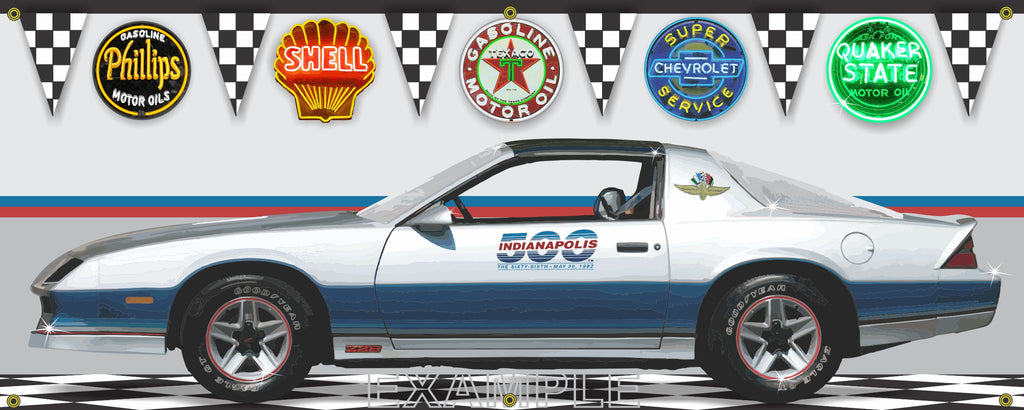The image depicts a pristine silver car resembling a Trans Am or an early 80s/90s Camaro parked on a checkered floor. The vehicle features a prominent blue stripe running along its lower body and displays "Indianapolis 500" text on its driver-side door, indicating its race car status. The car's condition is immaculate, with windows rolled down and tires that include a distinctive red trim around the rims. It is situated inside a well-lit display room.

The background includes a white wall adorned with a red stripe beneath a blue stripe. Above these stripes, a series of triangular checkered flags are positioned, interspersed with various vintage gasoline and motor oil round signs. These signs include a bright green "Quaker State," a blue "Super Service Chevrolet," a red "Phillips Motor Oil" with a black and gold accent, a yellow "Shell" shaped like a shell with red text, and a red Texaco star in a banner. The composition of the image, with its color contrasts and detailed signage, evokes a nostalgic feeling tied to the Indy 500 racing culture.